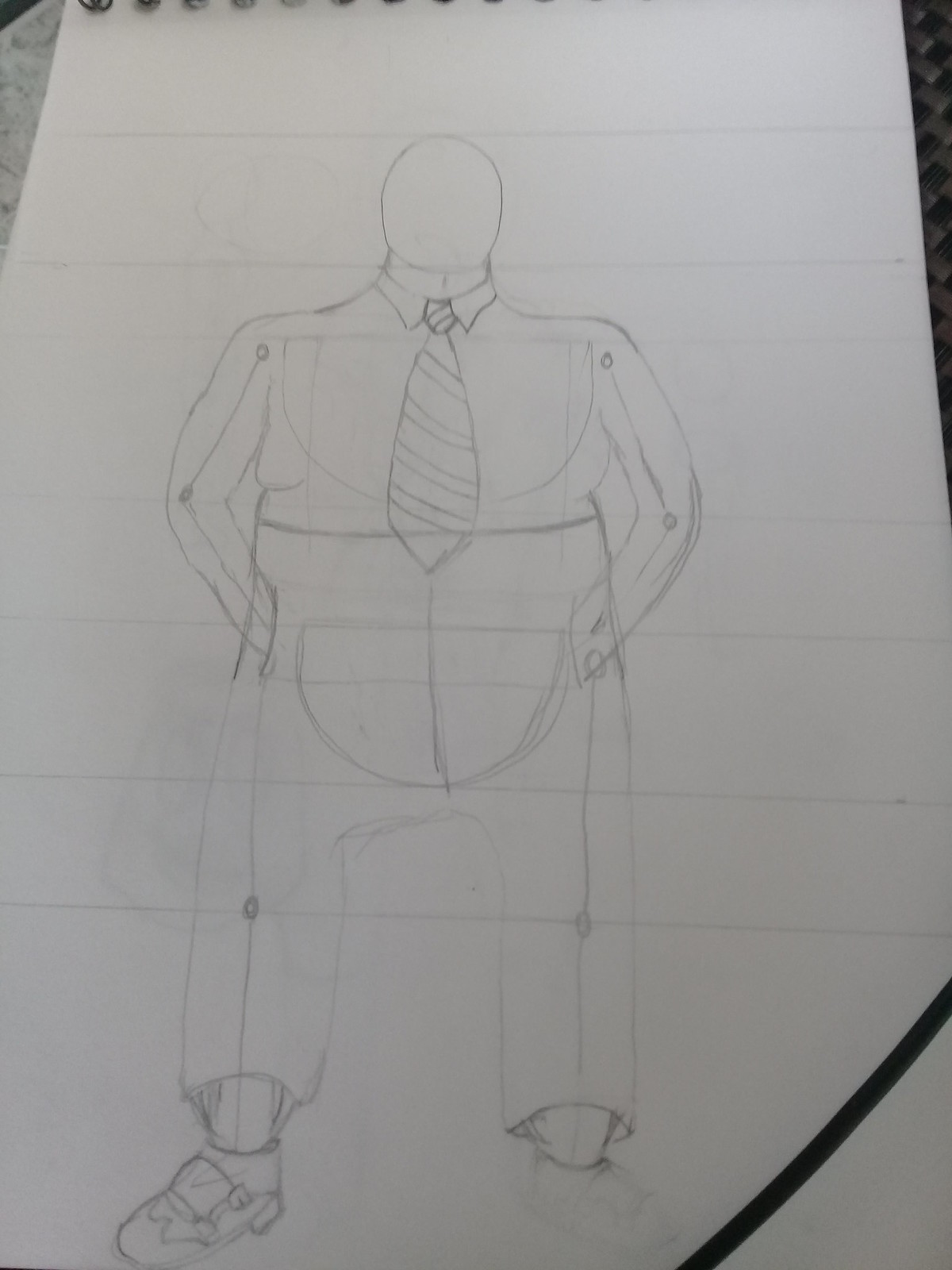A detailed wireframe diagram of a human figure is rendered on a white background. The figure is composed of numerous intersecting lines forming rectangles that outline the human body's structure from head to toe. Key anatomical points are highlighted, including the head, shoulder joints, elbow joints, wrist joints, knee joints, and ankle joints. The wireframe figure is dressed in pants, indicated by vertical and horizontal lines, and is also wearing a tie with curved lines suggesting its texture. The shoes, appearing as if they might have buckles, contrast with the legs that extend down to the feet at the bottom of the figure. The detailed wireframe illustrates both the skeletal framework and the clothing elements of the person.